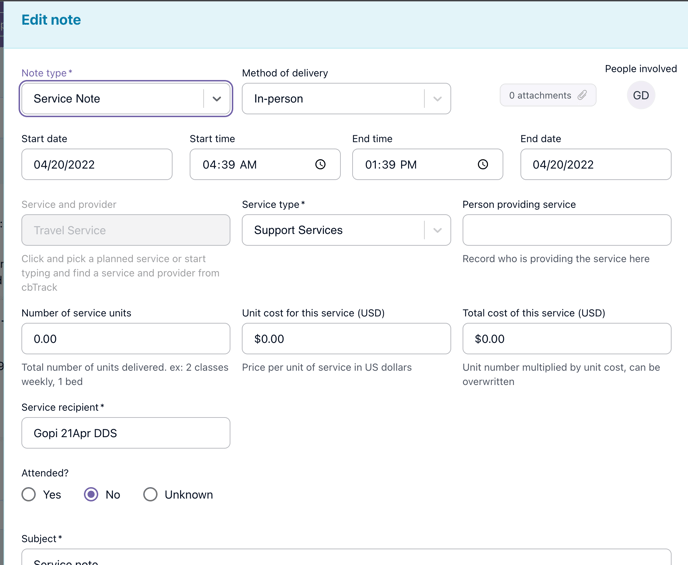This screenshot captures an application used for tracking detailed information about a service note. The user interface design features a light blue header strip at the top displaying the title "Edit Note" in blue text. The page is structured with multiple text boxes and drop-down menus for data entry.

- **Note Type**: The first text box is labeled "Note Type" and is currently selected, highlighted in purple, showing the option "Service Note" with a drop-down arrow for other choices.
- **Method of Delivery**: Adjacent to the Note Type, this field is displaying "In Person" indicating how the service was delivered.
- **Attachments**: There are no current attachments, but an option to add one is available through a clickable button.
- **People Involved**: This section shows a grey circle icon with the initials "GD," which could represent either a username or another identifier.

In the subsequent row:
- **Start Date**: Set to "04/20/2022" (April 20th, 2022).
- **Start Time**: Listed as "04:39 AM."
- **End Time**: Displayed as "01:39 PM."
- **End Date**: Also marked as "04/20/2022." This suggests that the service was delivered in-person between 4:39 AM and 1:39 PM on April 20th, 2022.

Further down:
- **Service and Provider**: This section is non-interactive and grayed out, reading "Travel Service." It offers guidance to "Click and pick a planned service or start typing to find a service and provider from CB Track," which implies CB Track is possibly the service management system in use.
- **Service Type**: Currently selected as "Support Services" from the drop-down menu.
- **Person Providing Service**: The box is empty, prompting to record the service provider's name.
- **Units of Service**: Listed as "0.00."
- **Unit Cost**: Shows "$0.00."
- **Total Cost**: Calculated as "$0.00."

Finally:
- **Service Recipient**: Entered as "GOPI 21 APR DDS," indicating the recipient's details and service date.
- **Attendance**: The attendance status presents options "yes," "no," or "unknown," with "no" currently selected.
  
This comprehensive form tracks various aspects of service delivery, including dates, times, involved parties, and financial details, offering a detailed review and management of service-related notes.